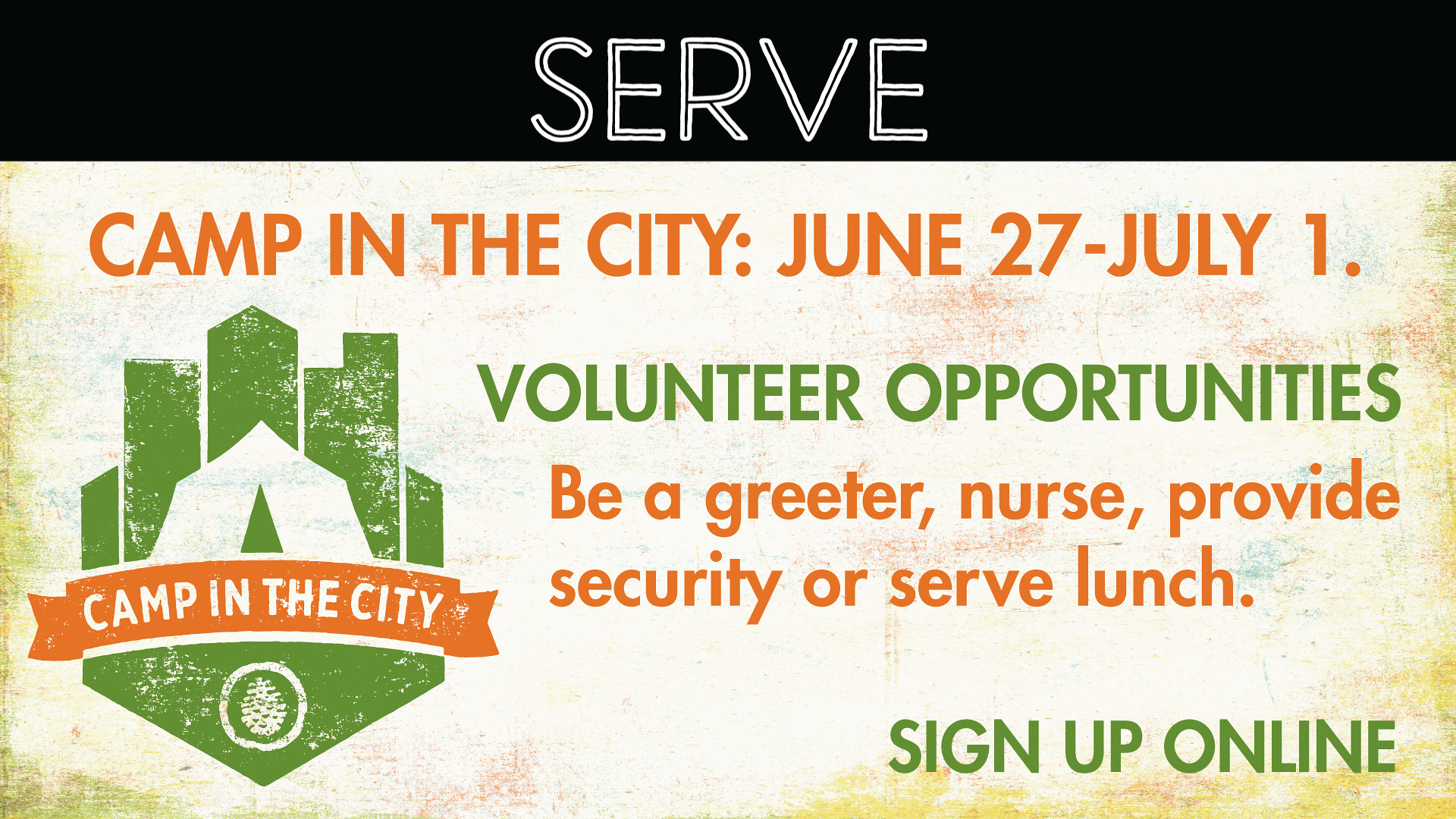The image is a digital poster with a textured background featuring shades of white, cream, red, and blue. A black bar spans the top quarter of the poster, with white text saying "SERVE," designed with a line through the middle of the letters to give a three-dimensional effect. The bottom portion of the poster has a cream-colored background with light brown smudges.

In uppercase orange text, it announces "CAMP IN THE CITY; JUNE 27 - JULY 1." Below this, in light green uppercase text, it lists "VOLUNTEER OPPORTUNITIES." The specific opportunities are detailed in orange text: "BEE A GREETER, NURSE, PROVIDE SECURITY, OR SERVE LUNCH."

At the very bottom left, in uppercase green text, it says, "SIGN UP ONLINE." Adjacent to this, there's a logo featuring the outline of tall skyscrapers in green, with a white tent above an orange banner that reads "CAMP IN THE CITY" in white text. The logo also includes a fur cone inside a circle, mounted on a badge-like triangle pointing downward.